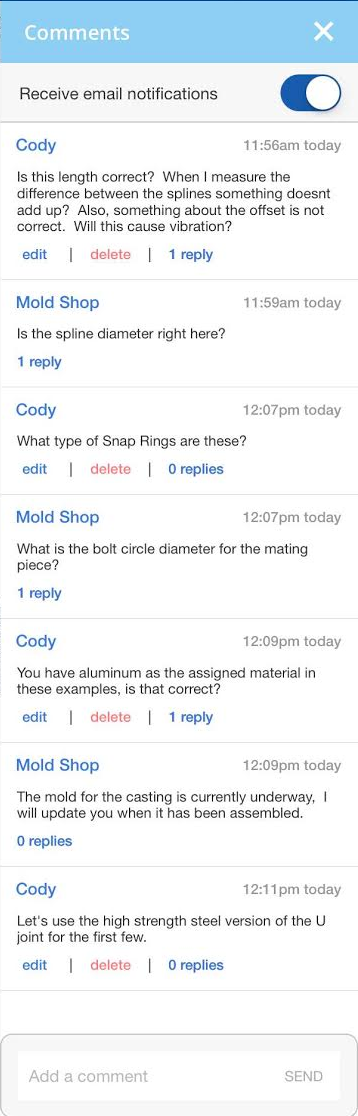**Screenshot Description**

The screenshot features an interface with a white background, containing two distinct sections for displaying information. At the top of the screen, a light blue bar runs horizontally. On the left side of this bar, the word "Comments" is displayed in white text, while a white "X" icon is positioned on the right. Directly below this blue bar is another horizontal bar, this one shaded in gray. It reads "Receive email notifications" with a blue toggle switch to the right; the toggle switch has a white circle indicating its active state.

The main content of the page is divided by vertical lines into different dialogue sections. Each section represents a conversation thread between various participants:
 
1. **Cody:**
   - Text: "Is this length correct when I measure the difference between the spine lines and something doesn’t add up? Also, something about the offset is not correct. Will this cause vibration?"
   - Options: "Edit" (in blue), "Delete" (in pink), "1 Reply" (in blue)

2. **Mold Shop:**
   - Text: "Is the spline diameter right here?"
    
3. **Cody:**
   - Text (in blue): "What type of snap rings are these?"

4. **Mold Shop:**
   - Text: "What is the bolt circle diameter for the mating piece?"

5. **Cody:**
   - Text: "You have aluminum as the assigned metal in these examples. Is that correct?"

6. **Mold Shop:**
   - Text: "The mold for the casting is currently underway. I will update you when it has been assembled."

7. **Cody:**
   - Text: "Let's use the high-strength steel version of the U-joint for the first few." 

Each text exchange is neatly separated, facilitating easy readability and follow-up actions on specific comments.